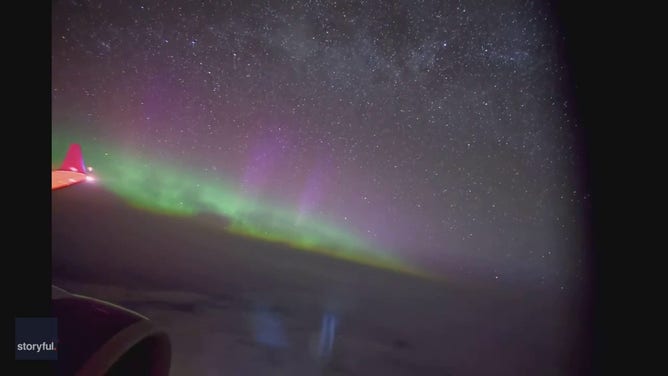The image, likely a color photograph or illustration, captures a night scene from the perspective of an airplane window. The Northern Lights, or aurora borealis, dominate the sky with a stunning display of green and purple hues, softly merging into each other and adorned by scattered twinkling stars. In the lower left corner, a small watermark in whitish grayish letters spells out "storyful," possibly indicating a brand name. Adding an intriguing twist to the scene, the lower left corner also includes part of the airplane's body and wing, which are tinged with a pink light. Notably, there is an unusual, distinctly unnatural feature on the left side of the image: an orange shape topped by a red triangle emitting small white glowing lights, hinting at an object or scene from a video game. The overall composition of the photo is very dark, accentuating the vibrant Northern Lights and the mysterious elements within the image.